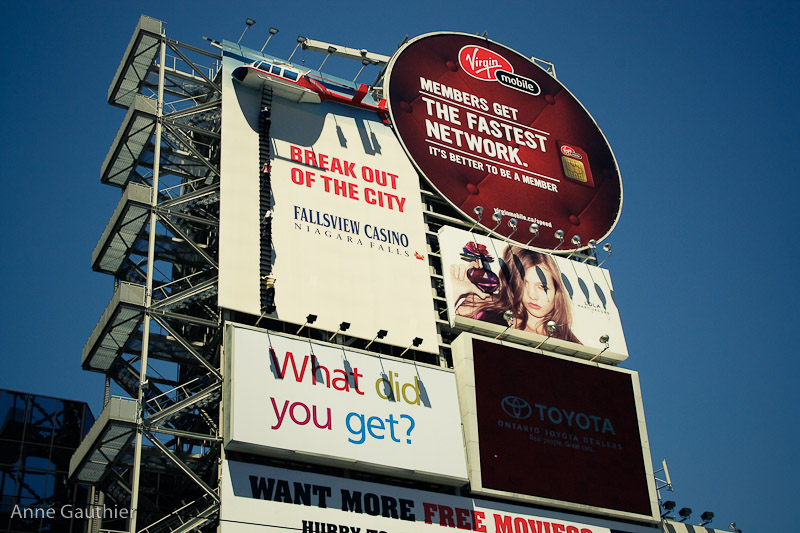The image captures the facade of a tall building adorned with various advertisements. On the left side of the building, multiple open flights of stairs ascend in a C-shape, indicating there are five levels. The building is surrounded by a bright blue sky, giving it an open-air appearance reminiscent of scaffolding or an arena scoreboard.

At the top right of the building, there is a large circular advertisement for Virgin Mobile with the slogan, "members get the fastest network. It's better to be a member." Below this, a poster features a woman's face, possibly advertising perfume, as there is a hint of a perfume bottle to the left of her image. Beneath this, another advertisement for Toyota is displayed, with a digital text that includes the name Ann Gunther in the bottom left corner.

On the left side of the structure, a distinct ad shows a helicopter with the phrase "break out of the city," accompanied by an image of people climbing a rescue ladder, indicating it's from Falls View Casino in Niagara Falls. Below that, there is a text-based advertisement where the words "what did you get?" are color-coded in red, olive green, magenta, and blue, respectively. Finally, an advertisement stretching across the width of the structure partially reads, "want more free movies?" although the complete text is not visible in the picture.